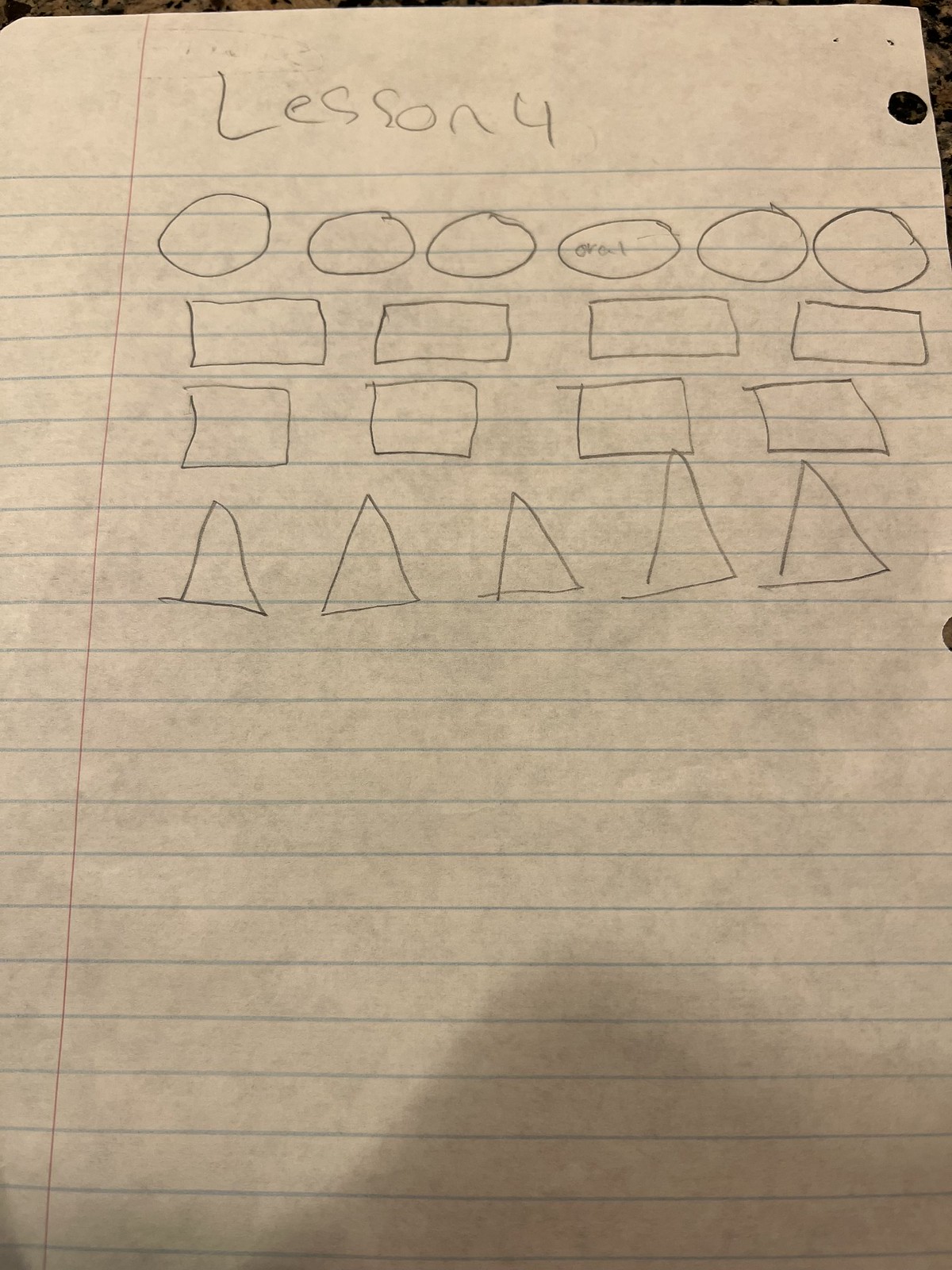This is a meticulously detailed pencil drawing on a sheet of standard white lined paper. The paper is oriented with the three hole punches on the right-hand side. A red vertical line marks the left margin, while evenly spaced blue horizontal lines traverse the entire page. 

At the top of the page, written in pencil, are the words "Lesson 4." Directly beneath this heading, six circles of varying sizes are arranged horizontally across the sheet. These circles range from perfectly round to more oval shapes. 

Positioned below the circles are four rectangles, also aligned horizontally. These rectangles differ in size and are irregularly spaced. 

Following the row of rectangles, four squares are horizontally spread across the page. Similar to the other shapes, the squares vary in both size and spacing.

At the bottom, five triangles are lined up horizontally. These triangles are also inconsistent in their dimensions. The first three triangles maintain a similar size, while the last two are notably taller. The fourth triangle even intersects with the lower right corner of the square directly above it, creating a visually intriguing overlap.